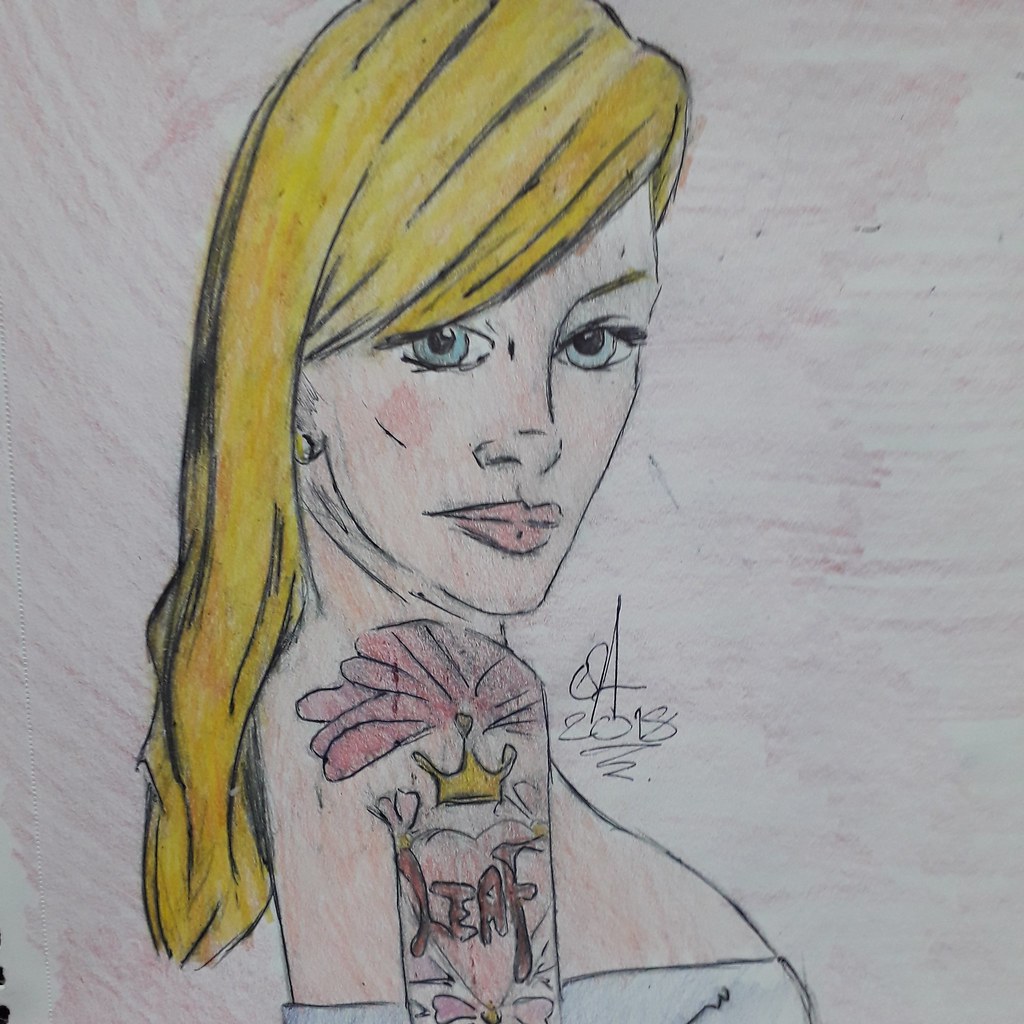This detailed drawing portrays a woman with her body oriented to the right, while her head is turned to face the viewer directly. Her right shoulder and arm are visible at the top of the image. Adorning her shoulder is a distinctive tattoo featuring a yellow crown embellished with what appears to be small red flowers. Beneath this crown, there is a heart inked with the word "LEAF" written across it in bold, capital letters. The woman has striking blonde hair and blue eyes, complemented by her pale skin, rosy cheeks, and pink lips. She is depicted wearing a light blue halter top or dress, which is visible towards the lower part of the drawing.